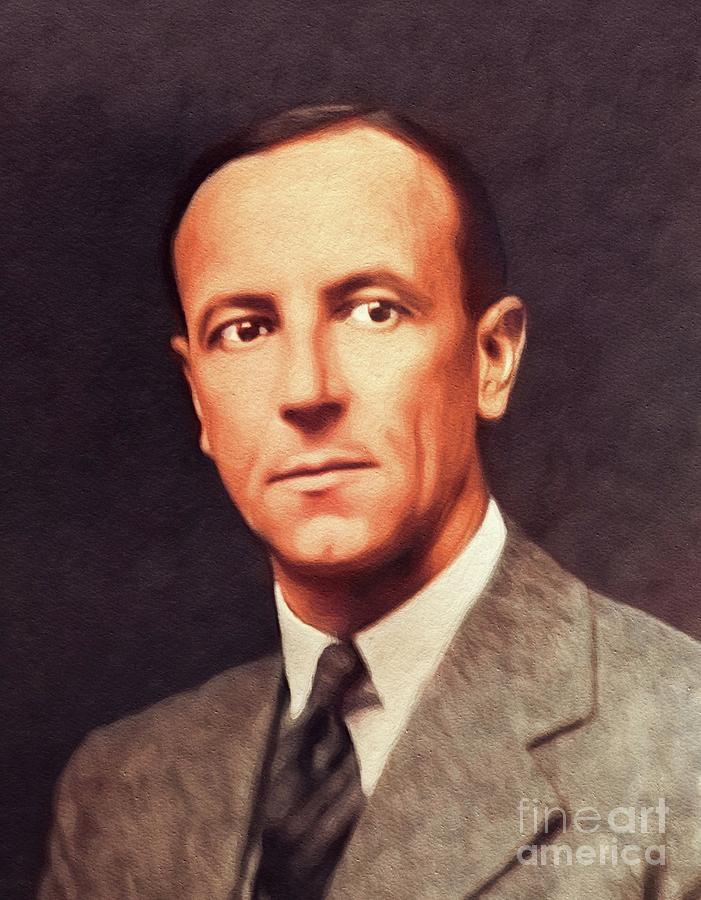This vintage portrait painting depicts an early middle-aged man with fair skin and a serious, thoughtful expression. Facing the viewer, his black eyes glance slightly to the right. He has short, neatly combed brown hair with a receding hairline and is dressed in a light gray suit, a white shirt, and a black and gray striped tie. The painting is rendered with a slightly blurred effect, possibly due to brush strokes or a photographic filter. The background is a modeled blend of light and dark gray, resembling a photographer's studio backdrop. The overall mood of the image hints at a dated period, possibly indicated by the man's attire and the style of the portrait. A watermark reading "Fine Art America" is present at the bottom right corner.